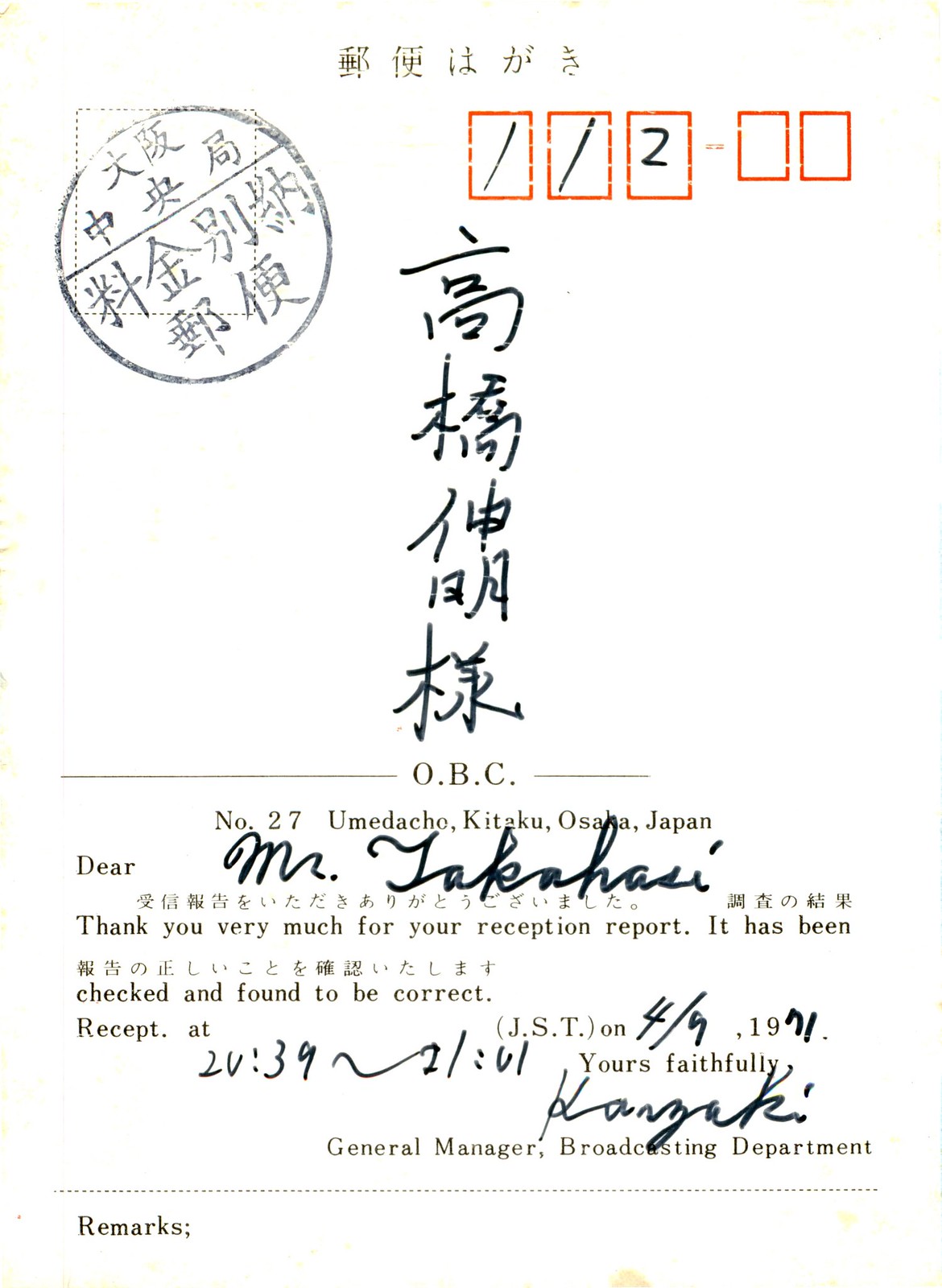The color image depicts an old Japanese receipt primarily written in Japanese. At the top, there are several blocks with handwritten Japanese characters and the number 112. The receipt, addressed from OBC, Number 27, Umadako, Kitaku, Osaka, Japan, acknowledges a reception report. It reads: "Dear Mr. Takahashi, thank you very much for your reception report. It has been checked and found to be correct. Receipt at 2039-2101 on 4-9-1971." The letter is signed by Hazaki, the General Manager of the Broadcasting Department. There is a section labeled "Remarks" at the bottom, which is left blank.